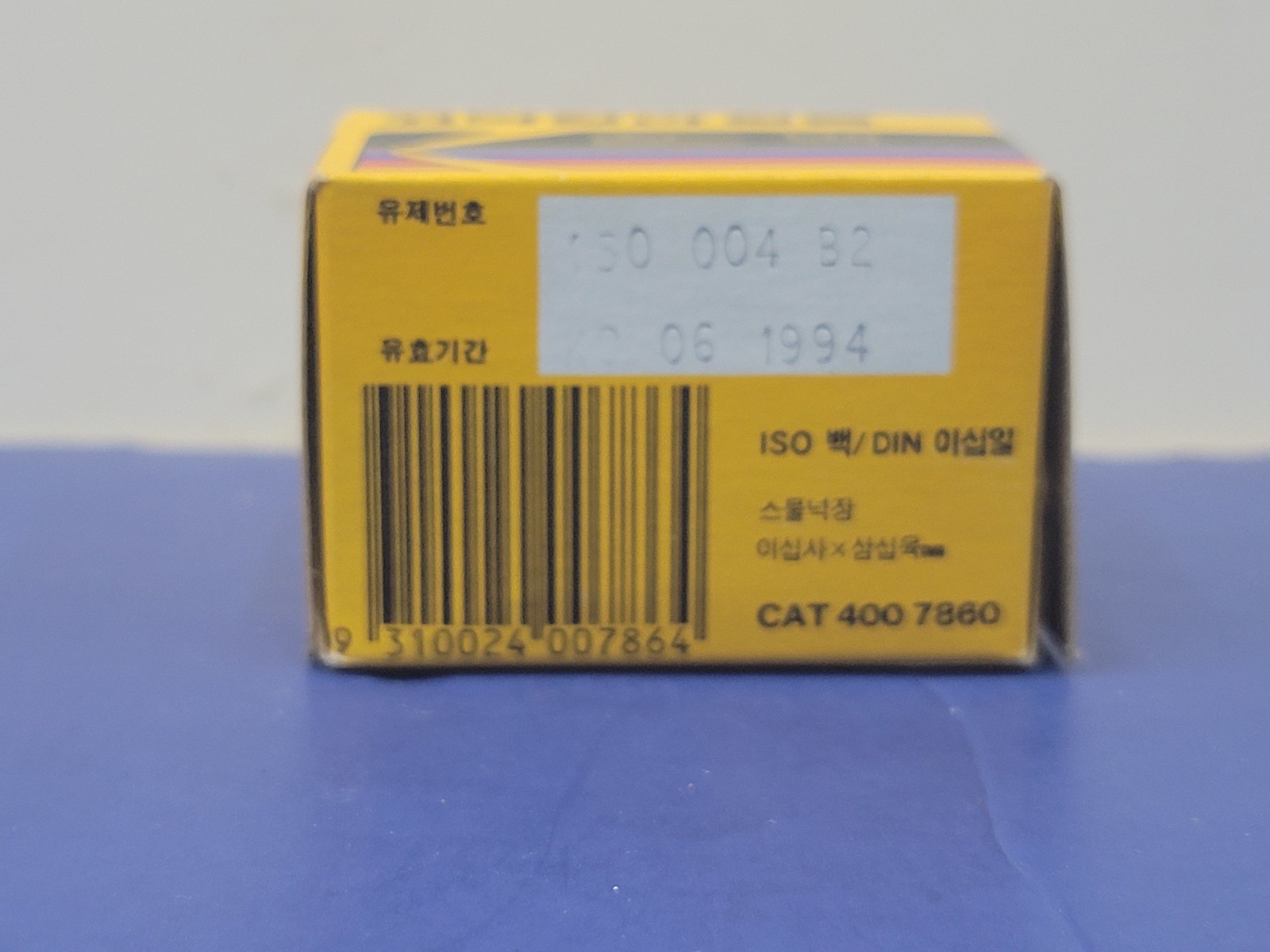Photograph of a yellow box prominently labeled "CAT-400-7860-ISO-DIN" against a blue surface, with a white background wall. The box features Chinese text on the left side and a barcode situated at the bottom left corner. The date "06-1994" is clearly visible, adding a sense of time to the image.